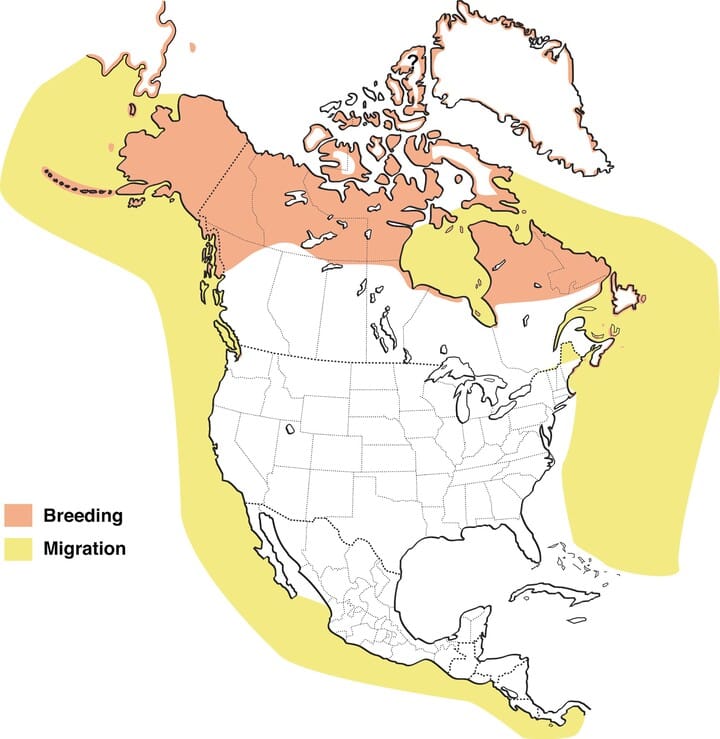The image depicts a detailed map of North America with specific regions color-coded to signify the behavior of a species, likely a bird or insect. The Pacific Ocean and parts of the Atlantic Ocean are prominently shaded in yellow, indicating migration routes. In addition, the yellow migration paths stretch from southern South America up through coastal regions of Alaska and Canada, also covering the area from the Great Lakes straight down to the side of Florida. Mainland United States remains uncolored, except for Maine, which is marked yellow. Meanwhile, the northern parts of Canada and parts of Greenland are distinctly colored in red, denoting breeding grounds. The left side of the image features a legend clarifying that red represents breeding areas and yellow indicates migration zones. This detailed color-coding provides insight into the species' breeding and migration patterns, with oceanic pathways and extensive northern territories covered.